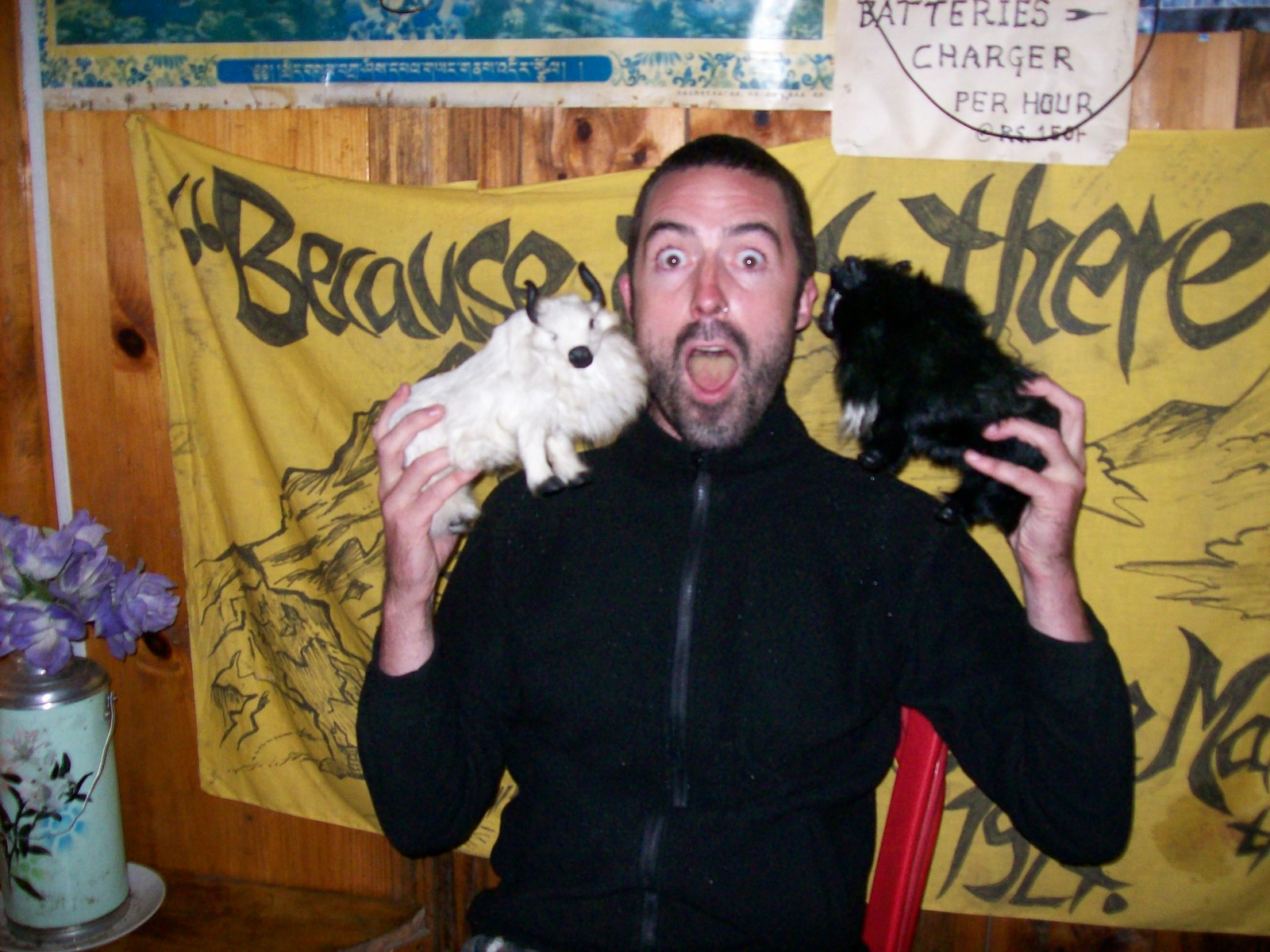The photograph captures an indoor setting featuring a central figure—a man with short brown hair, wide eyes, and a shocked expression directed at the camera. He is wearing a black long-sleeve zip-up jacket and holding two stuffed animals with horns, one white and one black, against his face. The background includes a wood-paneled wall adorned with a yellow sheet or fabric, a partial sign reading "batteries charger per hour," and a floral pot or tin with purple flowers in the bottom left corner. The scene is vibrant with various colors including purple, white, green, light blue, blue, black, red, yellow, and brown. The image conveys a somewhat playful yet perplexed atmosphere, possibly inside someone's home or a place of business.